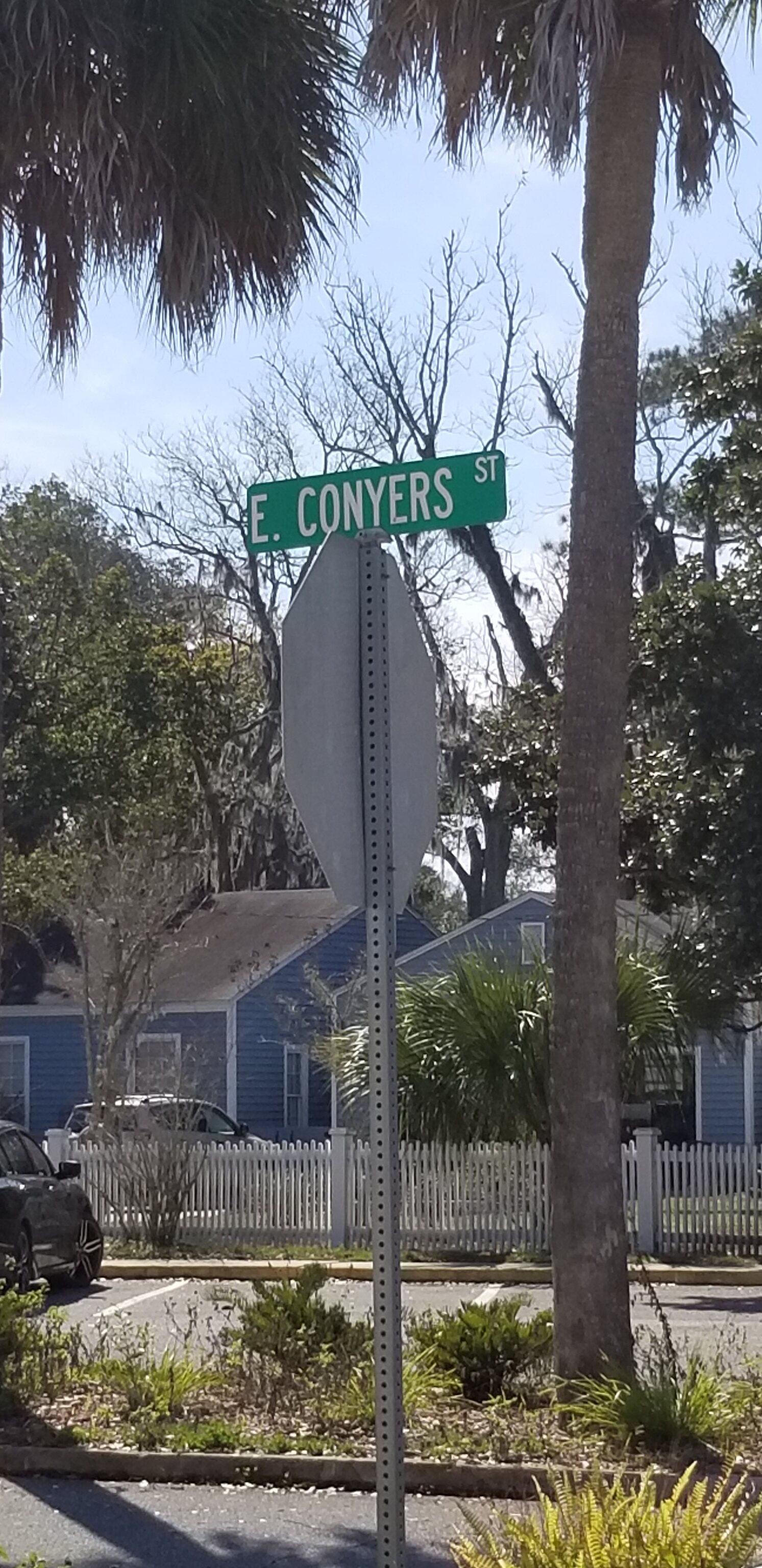A daytime photograph captures a detailed streetscape on East Conyers Street. The most prominent feature is the green street sign with white lettering mounted atop a metal post, indicating "East Conyers Street." In the background, a charming blue house with white trim and a glimpse of a gray roof stands out, partially obscured by a lush green tree and a classic white picket fence. A light-colored car is parked in front of the house, while a darker vehicle is visible beyond the fence, suggesting a parking lot. The foreground features patches of green plants, adding a touch of nature to the urban scene.